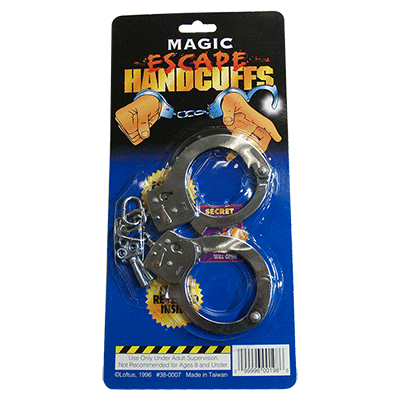The image features a product package for toy handcuffs against a plain white background. The toy handcuffs are encased in a clear plastic protective barrier and secured to a vertical package. The top of the package has a black background displaying the text "MAGIC ESCAPE HANDCUFFS" in all caps, with "MAGIC" in white, "ESCAPE" in orange, and "HANDCUFFS" in yellow. Below this title is a cartoon illustration of a pair of hands in handcuffs, with one handcuff open, indicating escape.

The package itself transitions from black at the top to blue towards the bottom. The handcuffs, made of dull silver metal, are front and center in the plastic casing, along with a small key. A white rectangular label containing a barcode is positioned at the lower right corner. On the lower left, there is a diagonal striped rectangle with alternating yellow and black stripes, and below it, a safety warning reads: "Use only under adult supervision, not recommended for ages 8 and under."

There is also some additional writing and numbers towards the bottom, indicating that the product was made in Taiwan, although these details are partially obscured by the handcuffs. The package includes a cutout hole at the top for hanging on store racks, completing its retail presentation.